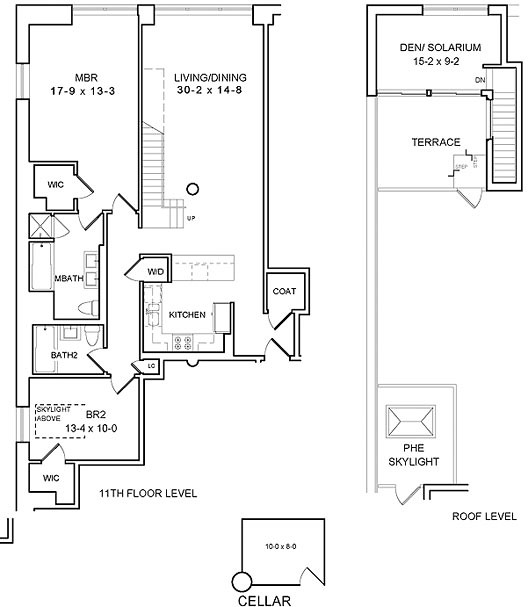**Detailed House Blueprint Description:**

The blueprint image depicts a house layout rendered in black lines on a pure white background. It's a scanned copy of the original blueprint. 

**Lower Section:**

- **Bottom Center:** A small square labeled "10 x 8" with the word "Cellar" in black font beneath it. Above this label, towards the left, the blueprint reads "11th floor level."
  
- **Lower Left:** 
  - A compact room marked "WIC" (Walk-In Closet).
  - Directly above the WIC is a square labeled "BR2" (Second Bedroom) with dimensions of "13.4 x 10." This room features a small box labeled "Skylight" towards the top. Additionally, there's a door on the left wall of this bedroom.

- **Above the Second Bedroom:**
  - A hallway extending horizontally.
  - To the left of the hallway is a small square marked "Bath 2" (Second Bathroom).
  - Above "Bath 2" lies a larger square labeled "Main Bath" (Main Bathroom).

**Right Section:**

- **Opposite the Hallway and Bathrooms:**
  - The "Kitchen" is situated, forming a central part of the layout.

- **Above the Kitchen:**
  - The "Main Bedroom" and the "Living/Dining Area" occupy prominent spaces.

- **Far Right Side of the Blueprint:**
  - The notation "Roof Level" appears.
  - A square labeled "Den."
  - Adjacent to it is a square for the "Terrace."
  - Another square labeled "Skylight" completes this section.

Overall, the blueprint carefully details the arrangement and dimensions of the various rooms and features in the house, providing a comprehensive layout of the 11th-floor level.